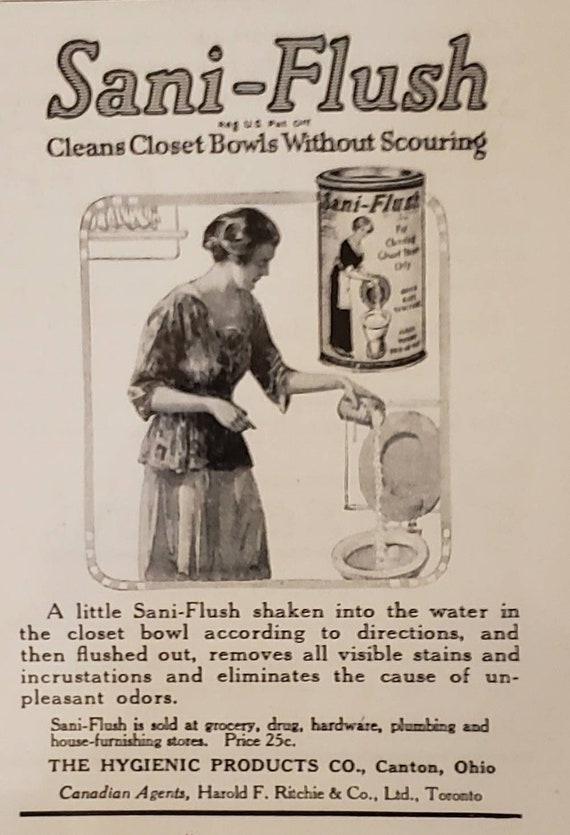This vintage, early 1900s-style advertisement for Sani Flush, printed in monochrome tones reminiscent of old newsprint, headlines with "Sani Flush: Cleans Closet Bowls Without Scouring." The central image showcases a woman in attire from the 1920s to 1950s, pouring a powder from a tin can into an open toilet bowl. Positioned above the toilet is a can of Sani Flush, featuring matching artwork. The caption under the image reads: "A little Sani Flush shaken into the water in the closet bowl according to directions and then flushed out, removes all visible stains and incrustations and eliminates the cause of unpleasant odors." Below, the advertisement lists the product's availability at grocery, drug, hardware, plumbing, and house furnishing stores for 25 cents. The Hygienic Products Company, Canton, Ohio, is credited as the manufacturer, with Canadian distribution by Harold F. Ritchie and Company, Limited, Toronto.